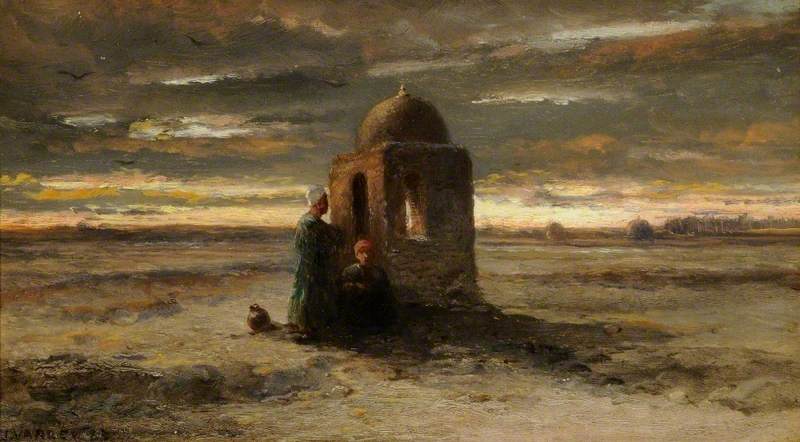This painting depicts two individuals beside a small, square, stone structure with a dome on top, reminiscent of an old toll booth or a modest Islamic building. The structure, featuring small windows and a tiny doorway, stands in the middle of a stark, flat landscape. The barren ground, a mix of brown hues, tans, reds, and dark grays, suggests a desolate or desert environment. The sky, with its rough texture and blend of brown, dark brown, white, greenish, and yellow tones, is illuminated by the golden and red hues of a setting sun, adding a dramatic backdrop to the scene.

In the middle ground, two figures can be seen. One, a man sitting down, wears a red hat and dark clothing. Beside him stands a person wearing a white scarf and a dark green dress. The minimalistic landscape in the far background features a faint building or structure and a tree line.

Birds are scattered in the upper left portion of the painting, adding life to the otherwise barren scene. The overall atmosphere of the artwork combines earthy tones and a dramatic sky, emphasizing the isolation and simplicity of the setting and its inhabitants.